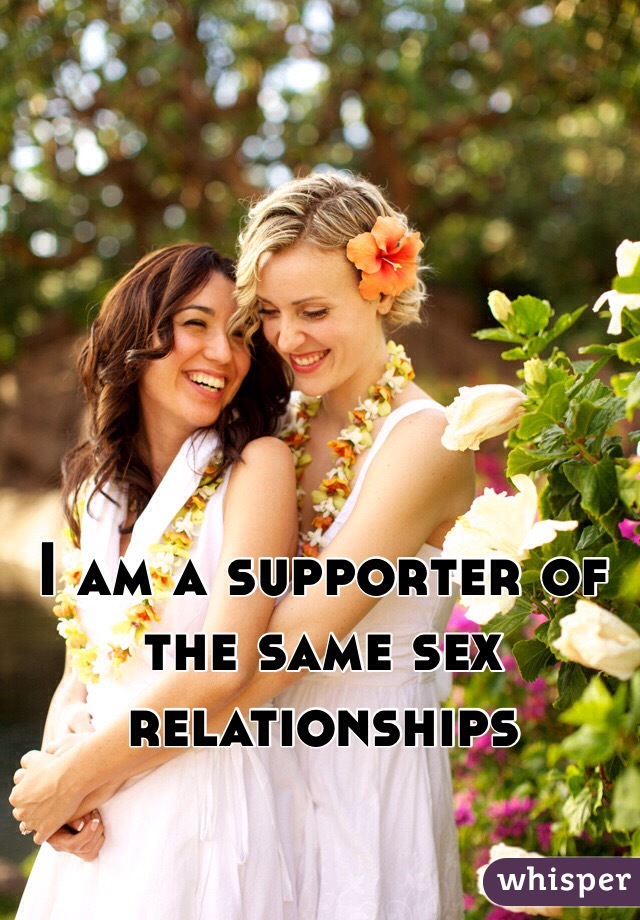In the center of the image, bold capitalized black letters spell out the title: "I AM A SUPPORTER OF SAME-SEX RELATIONSHIPS." Surrounding this text, a tender moment is captured between two women dressed in elegant white dresses, each adorned with a flower lei around their necks. The woman in front has long, wavy brown hair and gazes back affectionately at her partner. Standing behind her, a slightly taller woman with golden brown hair, accented with a flower above her ear, embraces her from behind. Their hands interlock gently, symbolizing their bond. Both women are smiling, their expressions filled with warmth and love. To the right, the image is adorned with lush green plants interspersed with delicate purple flowers, adding a touch of natural beauty to the scene. At the bottom of the image, the word "whisper" is subtly included.